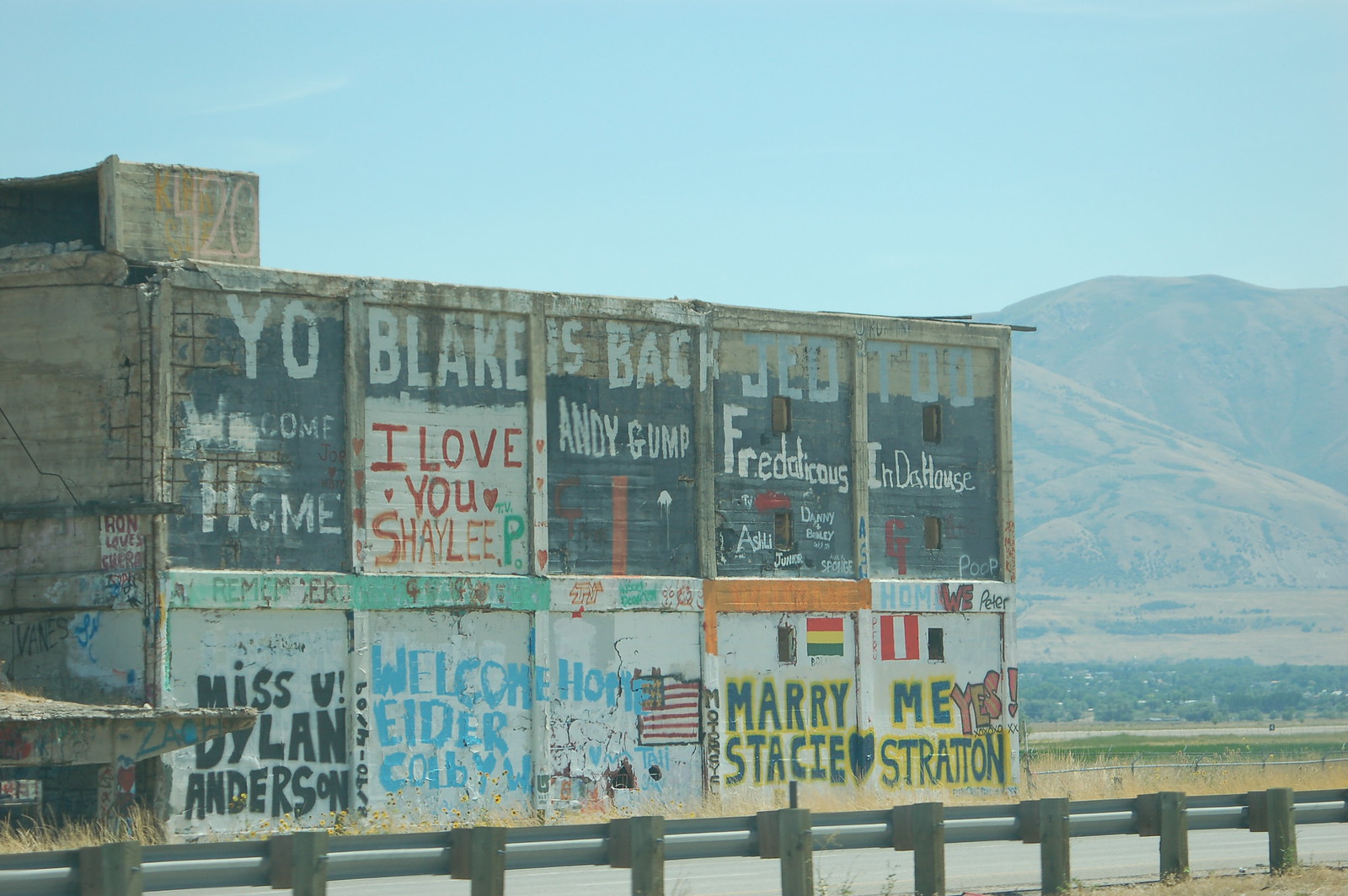In the image, there is an imposing, gray building structure situated behind a railing adorned with a series of messages. Starting from the top-left corner, the messages read: "Yo, welcome home," followed by "Blake, I love you," and "Shea sleep." Further to the right, the railing displays "back, Andy Gump," with "J.E.D." encircled by more writing. Next comes "Todd in the house," followed by "Miss You, Dylan Anderson" below it. Continuing to the right, the text reads "welcome, Elder Colby," with the subsequent message stating "home" alongside an American flag. Moving further, there is a message that reads "Mary Stacey" with a red, yellow, and green flag positioned in the top right corner. Adjacent to this is a flag featuring red, white, and red stripes and the message "me. Yes, Stratton."

The building and the railing with its varied messages comprise a visually striking and complex scene. The backgrounds of the messages are either white or blue. To the right of the scene, a picturesque mountainous landscape unfolds, enhancing the image with natural beauty. Above, a serene light blue sky stretches across the top of the image, creating a tranquil and balanced backdrop to the structured and message-laden foreground.